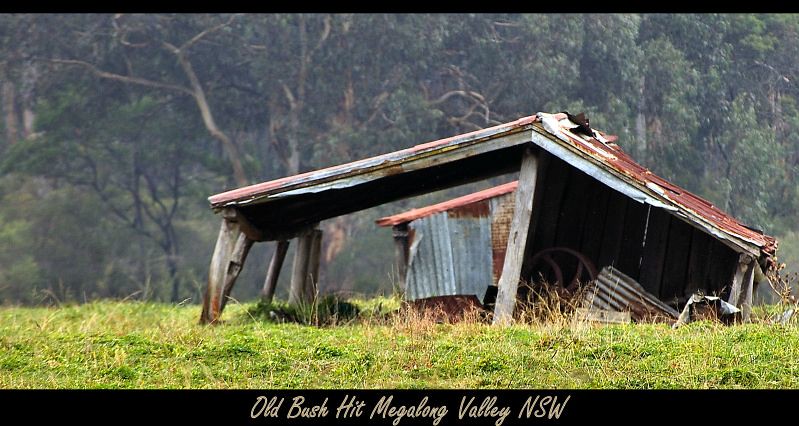In the foreground of this outdoor scene, an old, dilapidated farm building or shed struggles to remain upright amidst a field of long grass. The structure, predominantly made of rusted corrugated metal, tilts precariously to the right, its roof deteriorated and partially collapsed. The wooden beams and posts, once supportive, now barely hold up the remaining framework, revealing a wheel and other remnants inside. Behind this collapsing structure stands another building, partially clad in corrugated metal with evident rust and bend marks. Both buildings are situated in a sunny, open grassy field, with the backdrop of a dense forest stretching out in the distance. The scene is void of any human presence, emphasizing the sense of abandonment and decay. At the bottom of the image, in white font against a black border, reads the caption: "Old Bush Hit, Megalong Valley, NSW."